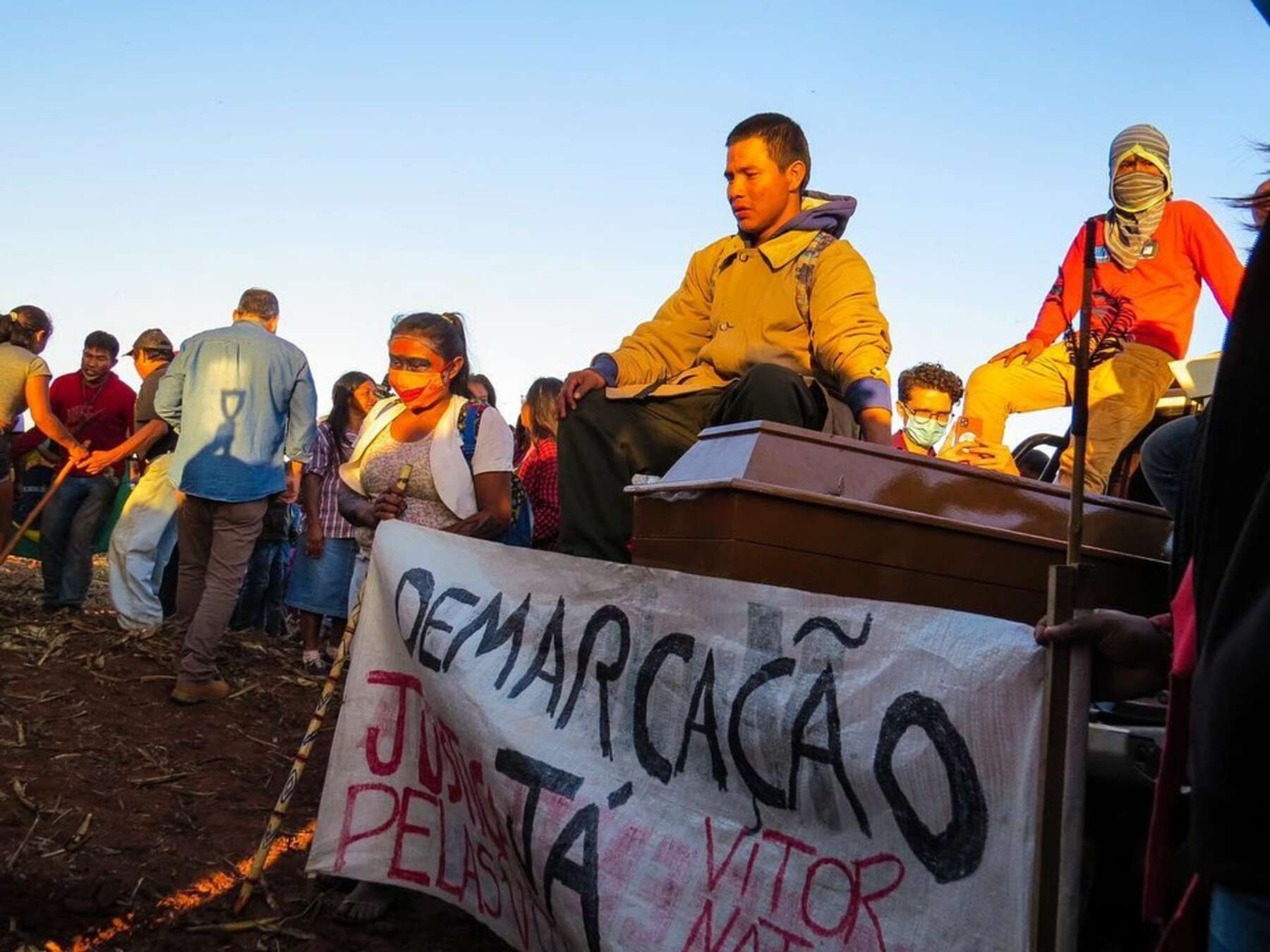The image depicts a scene under a light blue sky where a group of people, bundled up in heavy winter clothing, appear to be gathered for a protest. Prominent among the visuals are signs in Spanish. One sign reads "Justicia por Palacios," while another in black text reads "Dimar Kako," followed by "Vitor," which suggests a theme of victory. The people in the image seem cold and resolute, with some wearing masks and hats, and a few holding sticks. On the right side of the image, there is a shiny brown casket, which adds a poignant, somber element to the scene. A woman to the left, identifiable by her dark eye makeup and mask, adds to the intense atmosphere. Additionally, two individuals are seated on chairs, one in front of the other, further contributing to the intricate dynamics of this protest setting.